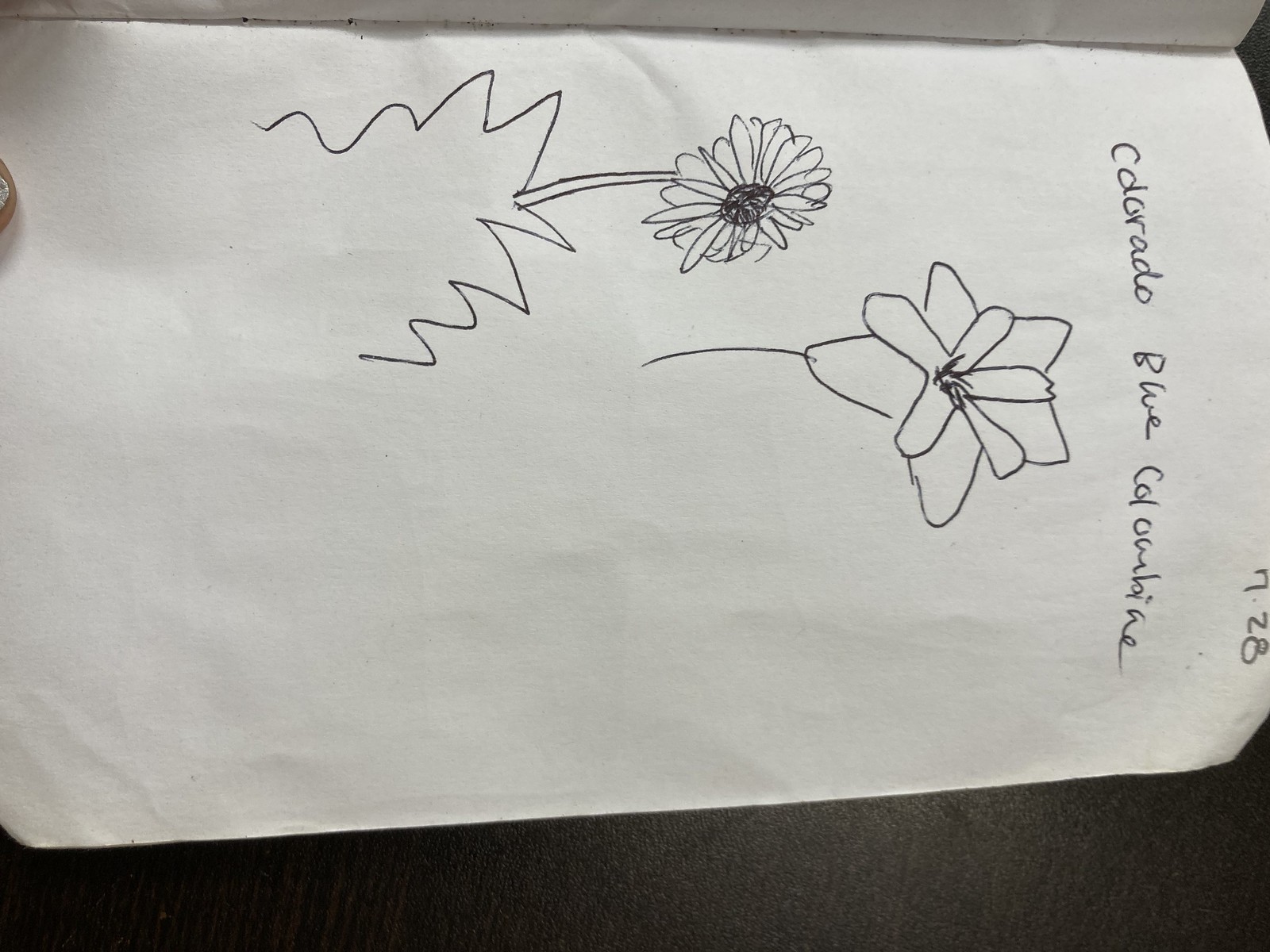This image features a white piece of paper placed on a dark brown wooden surface with visible black lines running through it. The paper is held by a person, whose finger and nail appear in the top left corner of the picture. The paper, oriented horizontally, bears a drawing of two flowers done in black ink. One flower, located towards the left, has uneven petals and a black center, appearing somewhat haphazardly sketched. The second flower, resembling a daisy with more detailed and symmetrical petals, a larger center, a stem, and a ground line, is situated more centrally. At the top of the paper, there is cursive handwriting in a foreign language, with the readable text "Colorado Blue Columbine" and the date "7-28" on the top right corner. The entire image is turned 90 degrees to the right, making the top of the paper appear as the right side.